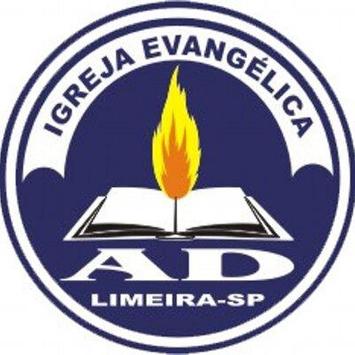The logo is circular with a dual blue circular outline around the edge. At the top of the emblem, a white circular arch prominently displays the words "IGREJA EVANGÉLICA" in blue, which is Portuguese for "Evangelical Church." The center of the logo features an open white book with blank pages, symbolizing the Bible, enclosed in an orange frame with a blue edge. Emanating from the book is a yellow and orange flame, adding a touch of artistic symbolism. Below the image of the book, the letters "A" and "D" are displayed in large capital letters. Further down, the text "LIMEIRA-SP" is printed in white, identifying a location in São Paulo, Brazil. The primary background color of the logo is a rich navy blue.